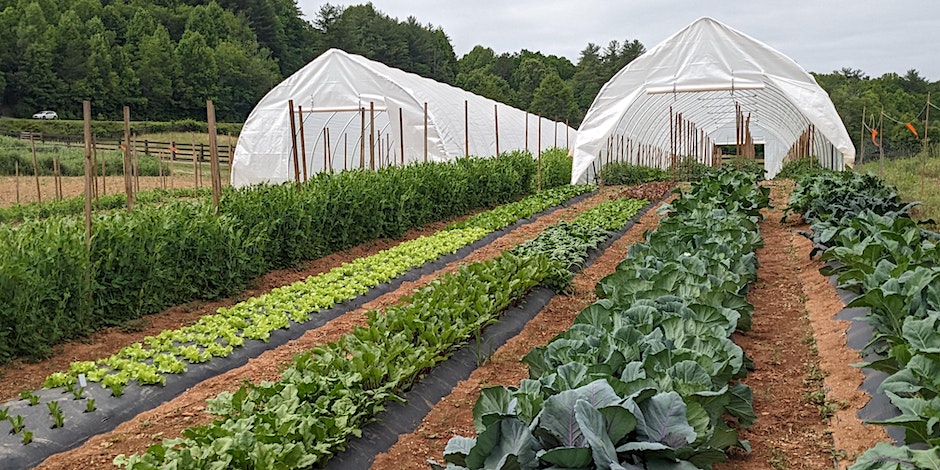The photograph captures a meticulously maintained farm with neat rows of various crops, predominantly cabbages, lettuces, and other leafy greens. There are five to six clear, straight lines of crops growing from fabric-covered rows. Flanking these rows are two long, white greenhouse structures, made from a transparent plastic film, suggesting a portable setup possibly used for vining plants like green beans or tomatoes. The greenhouses extend over the rows, allowing the plants to continue inside. In the background, a line of trees indicates a forest area, and a car can be seen on a road in the upper left corner of the image, adding to the rural setting.